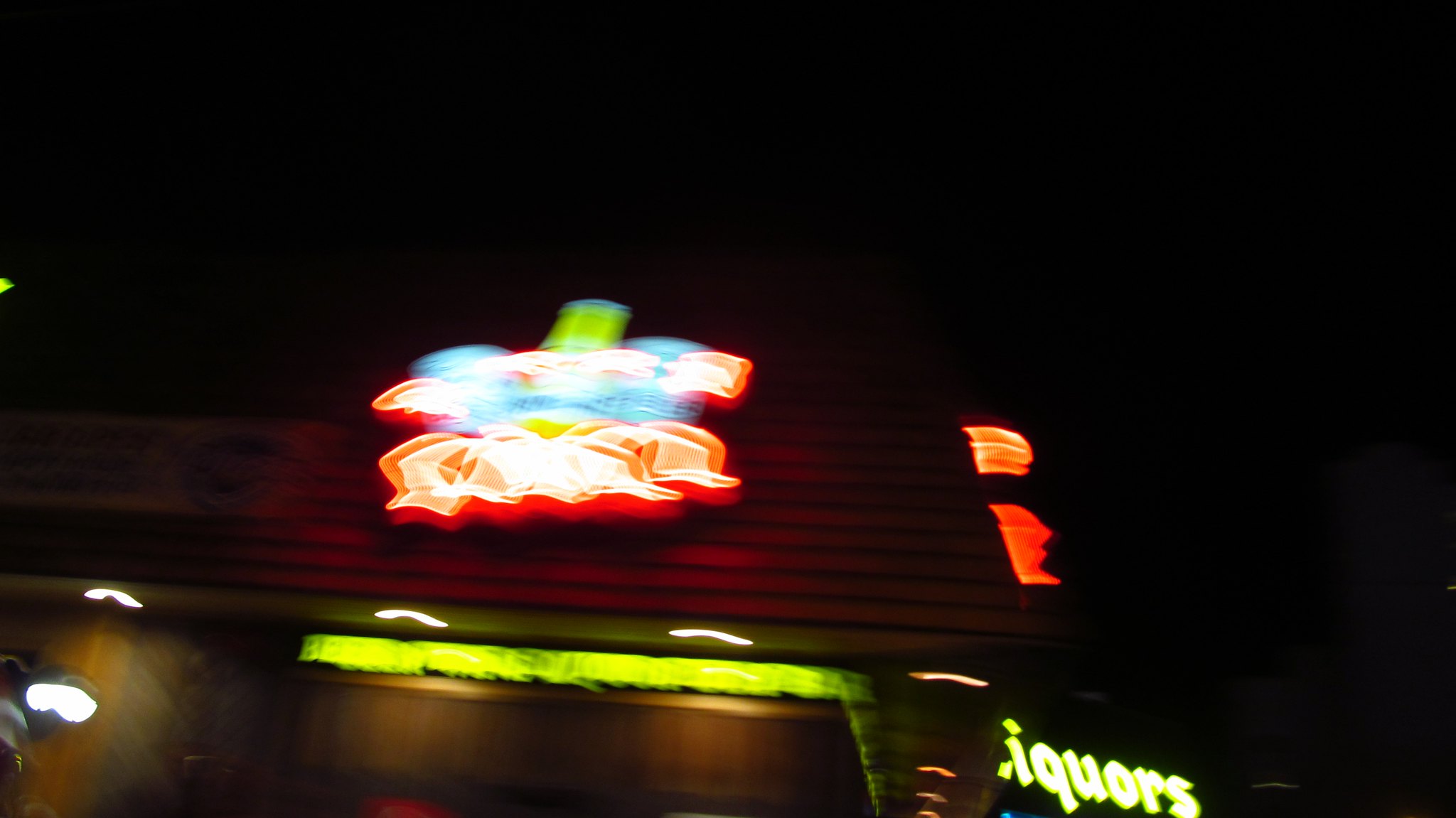In this color photograph taken at night, we see the outside of a business, viewed from an upward angle that emphasizes the dark nighttime sky. The top portion of the building features red, slatted paneling that wraps around the corner, illuminated by orange lighting. A prominent, albeit blurry, neon sign dominates the middle of the image; its unsteady glow suggests possible movement. The sign is a vibrant mix of lime green, blue, yellow, orange, and white, evoking the contents of a liquor bottle. Below this larger sign, there is another lime green light, and to its right, partially obscured but noticeable in white neon, the word "liquor" is displayed, with its initial "L" cut off. The neon's glow partially lights up what appears to be a doorway below, marked by additional yellow lighting strips and lime green illumination, contributing to the disorienting but colorful scene. The overall image is blurry, enhancing the sense of activity and the vibrancy of the various lights and colors.